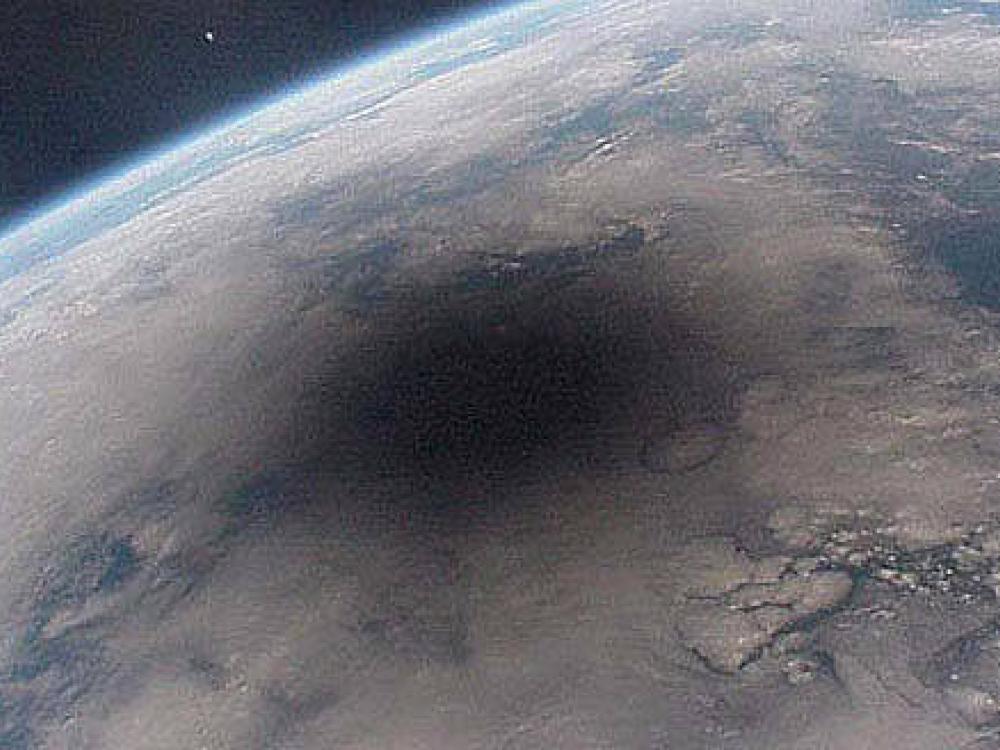This image captures a grainy view of a planet from space, closely resembling Earth or an Earth-like planet. The curvature of the planet is prominent in the upper left-hand corner, where the horizon is highlighted by a light blue hue indicating the atmosphere, set against the blackness of space. The reflection of sunlight in this region casts a gentle glow.

Dominating the center of the image is a striking, large dark spot. This spot, nearly jet black at its core, gradually fades into gray, blending with the surrounding landscape and cloud formations. The planet's surface showcases a mix of water bodies and brown earth, interspersed with various shades of brown and white specks, implying diverse surface conditions.

Adding to the celestial scenery is a solitary bright spot in the upper left, likely a star, reinforcing the cosmic setting. The planet's overall appearance is partly obscured by cloud or gas formations, making it difficult to discern detailed surface features, though hints of black swirls and rock-like structures suggest complex topography below.